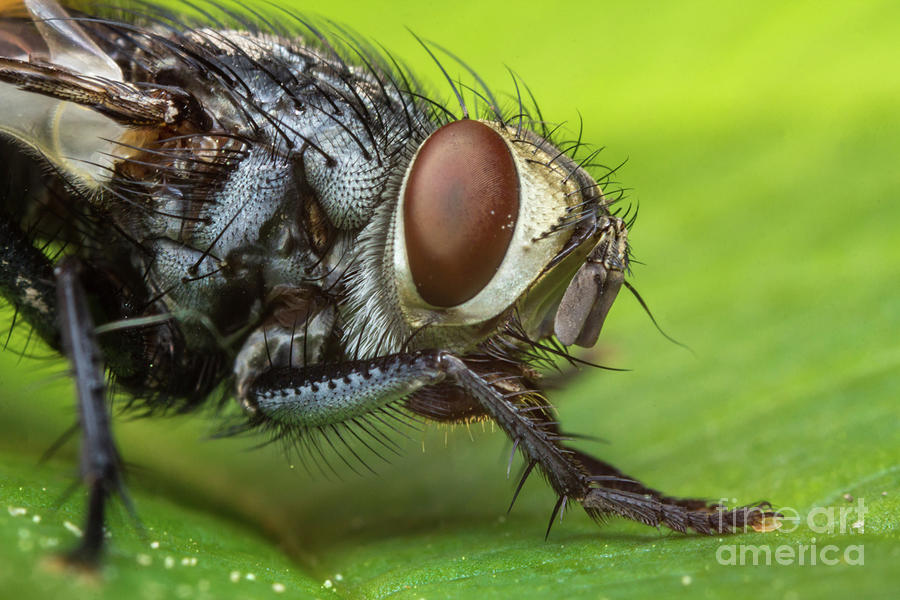This is an incredibly detailed, professional close-up photograph of what appears to be a common household fly. The fly's body, positioned from the left to the center of the image, is cut off towards the rear, focusing primarily on the torso and face. The intensity of the close-up reveals every minute feature, including coarse black hairs, spiny legs, and intricate pincers. The fly's eye, a dark reddish-brown oval, is particularly striking. Its transparent, clear wings can be seen with tinges of black and gray, and the image showcases the insect's multicolored body, embellished with shades of gold, white, gray, blue, red, and orange. Perched on a green leaf which is softly out of focus and adorned with tiny droplets of water, the fly's detailed portrait is both fascinating and unsettling. In the bottom right-hand corner, the white text reads "Fine Art America."